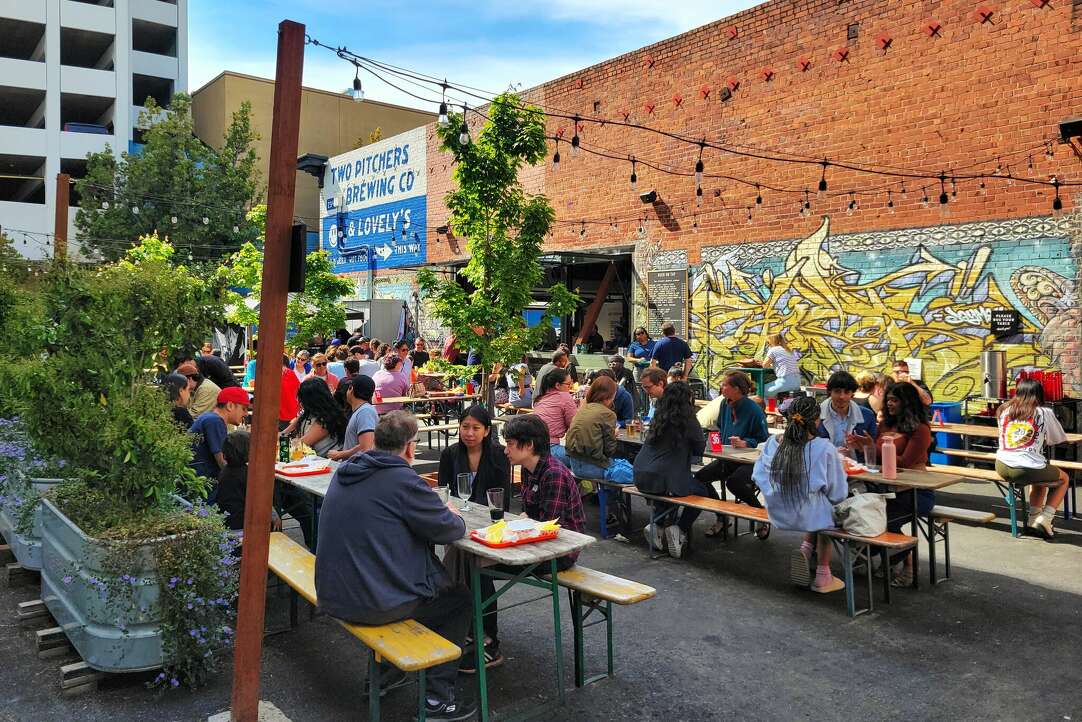In this vibrant outdoor scene, a group of adults is enjoying a sunny day at Two Pitchers Brewing Company, an outdoor restaurant aligned with a brewery. They are seated on long, cafeteria-style wooden benches and tables with green, metal legs, indulging in various snacks and treats, some accompanied by glass cups presumably filled with the brewery’s beverages. The backdrop features a reddish-orange brick building with a large, eye-catching sign that reads "Two Pitchers Brewing Co." in turquoise against a white background. Another phrase, "and lovelies," is displayed in a blue rectangle nearby. The right side of the building is adorned with a colorful mural in hues of yellow and blue, with squiggly lines that add a touch of artistic flair to the scene. Scattered around the area are potted trees and standing streetlights, contributing to the picturesque ambiance. In the distance, additional buildings in white and beige colors are visible. The overall setting, a likely company event or picnic, is filled with a lively atmosphere as people appear to be enjoying their meals and the beautiful weather.